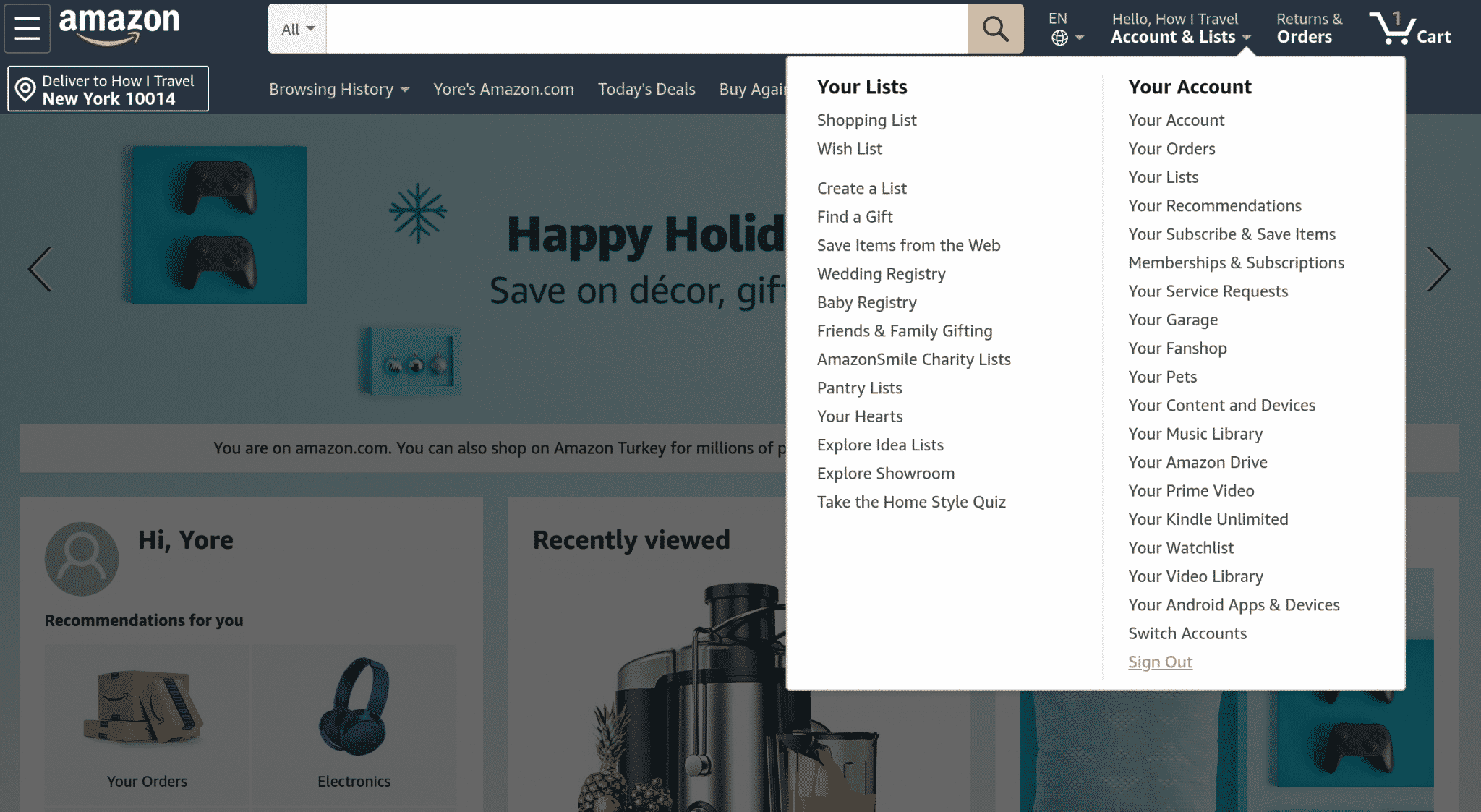This is a detailed screenshot from the Amazon.com mobile interface on someone's phone. In the upper left corner, the recognizable Amazon logo is prominently displayed, followed by a white search bar extending towards the center. Adjacent to the search bar are clickable links labeled "Account & Lists," "Returns & Orders," and a shopping cart icon in the upper right corner.

The user appears to have selected "Account & Lists," indicated by an arrow pointing towards it and an overlay box on the screen. This superimposed white box features black text and is divided into two main sections: 

On the left side, titled "Your Lists," it includes options like "Shopping List," "Wish List," and "Find a Gift," among others. 

On the right side is the "Your Account" section, which contains links such as "Your Orders," "Your Lists," and additional account-related options.

Behind this overlay, the Amazon homepage is partially visible, characterized by its blue and white color scheme. In the upper left corner, there are images of video game controllers. Below it, a seasonal message reads "Happy Holidays, Save on Decor," accompanied by a blue snowflake icon.

Towards the bottom left of the screen, a section greets the user with "Hi, [Username]" and offers "Recommendations for you," featuring images of Amazon boxes and headphones. In the bottom center, there's a "Recently Viewed" section displaying an item resembling a coffee machine.

The overall layout effectively combines the user's account management with a festive shopping experience.